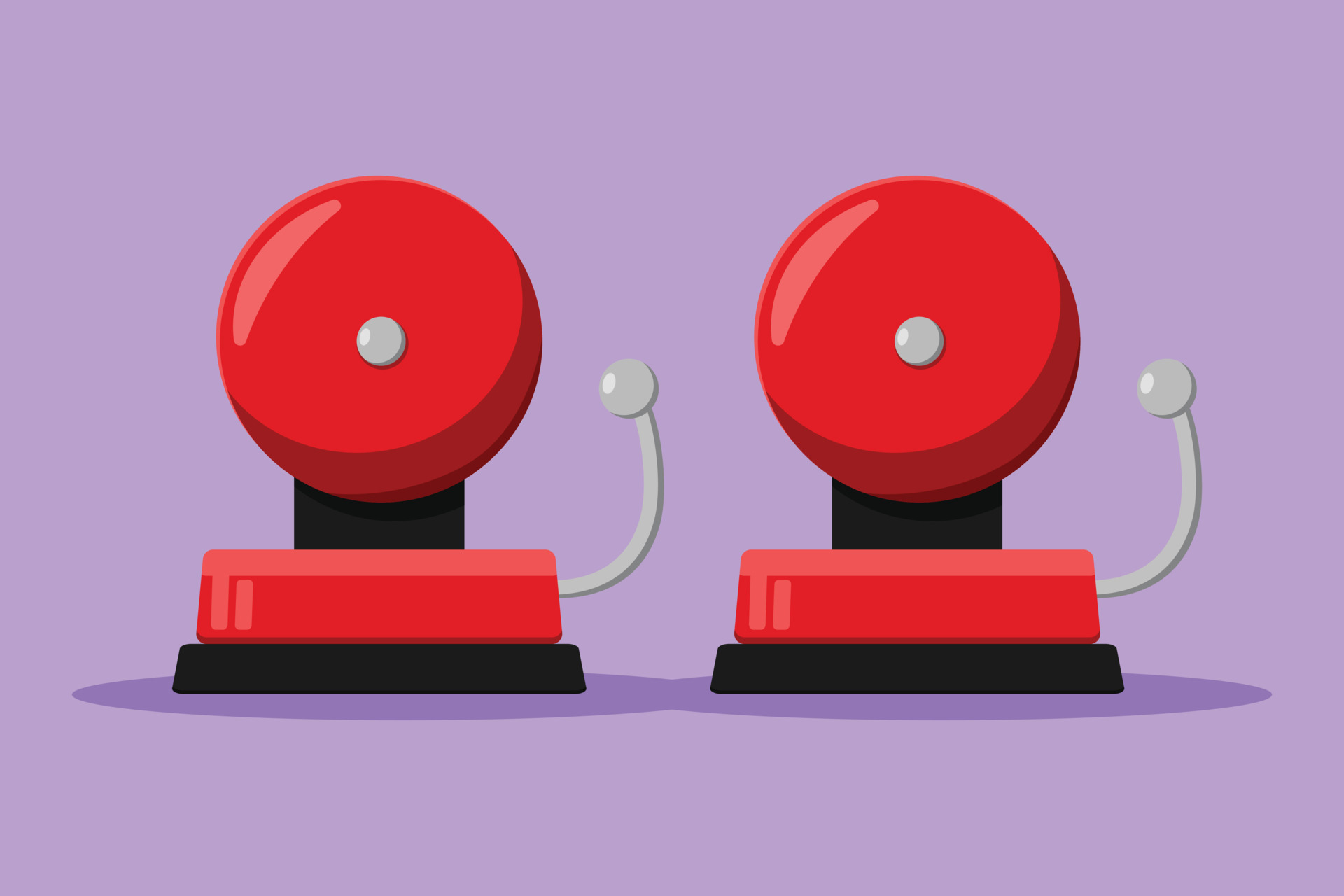The image depicts two identical red and black fire alarm bells sitting side by side against a light blue or lavender background. Each bell consists of a large red circle with a smaller gray circle at its center, connected to the main body by a black base that also houses a red bar on top. Extending to the right of each bell is a gray handle with a knob, intended to strike the red circle to produce a ringing noise. The bells cast dark blue shadows beneath them, adding depth to the scene. The overall style of the image suggests it could be either AI-generated or a detailed illustration.